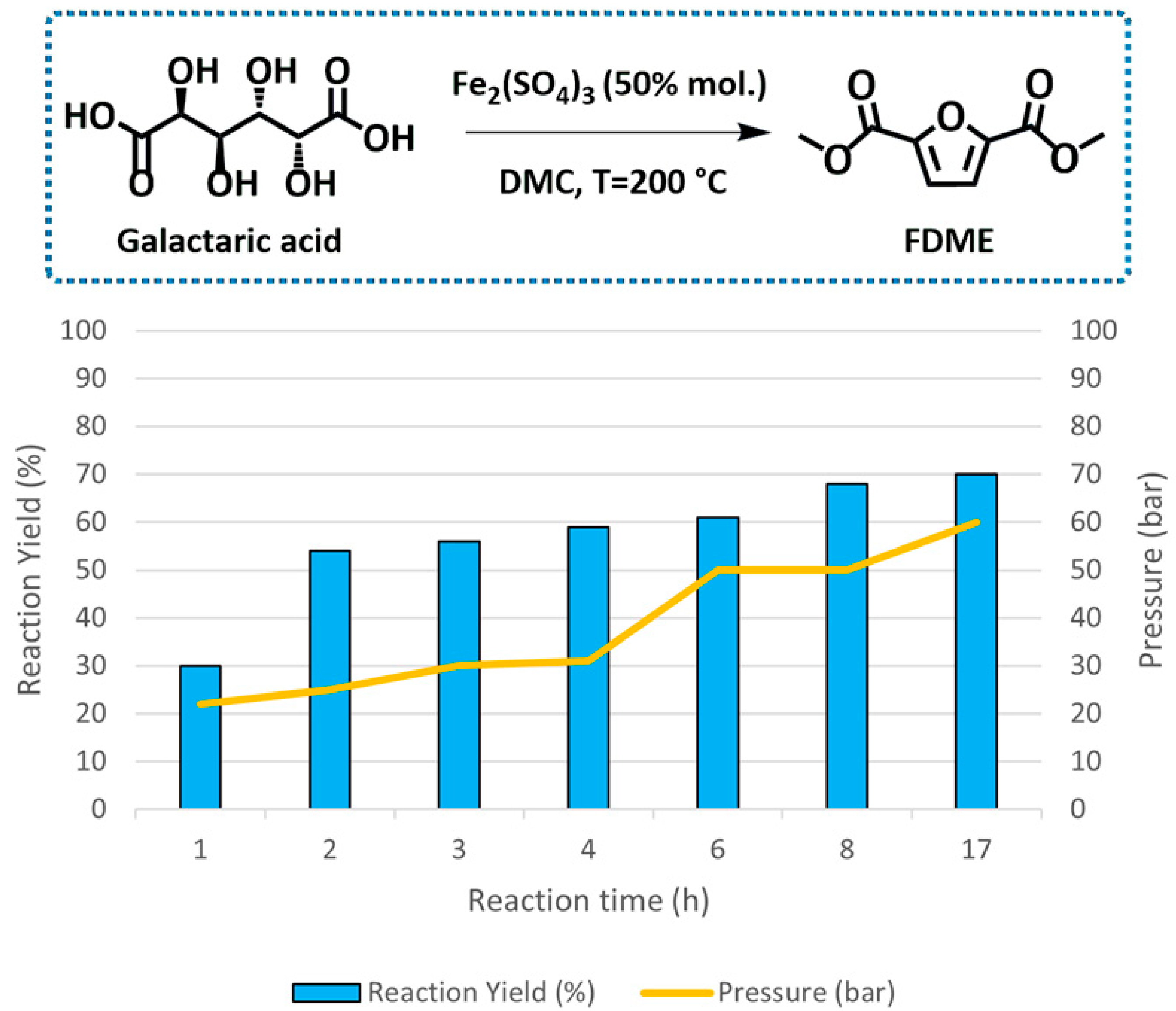The image depicts a combined line and bar chart representing an unspecified positive correlation over time. At the top of the chart is a rectangle spanning from left to right, outlined with a dotted blue line. Inside the rectangle on the left, there's an illustration of the molecular composition of Galactaric Acid, expressed as HO, O, OH, OH, OH, OH, O, OH. To the right of this molecular diagram, a black arrow points right, labeled with the chemical composition FE2, SO4, 3, 50% MOL, and the text DMC, T equals 200 degrees Celsius. Below this rectangle, the graph features a vertical line and bar chart with text labels indicating reaction time on the x-axis and reaction yield on the y-axis. The chart and captions are set against a white background, with blue color lines highlighting the data trends.